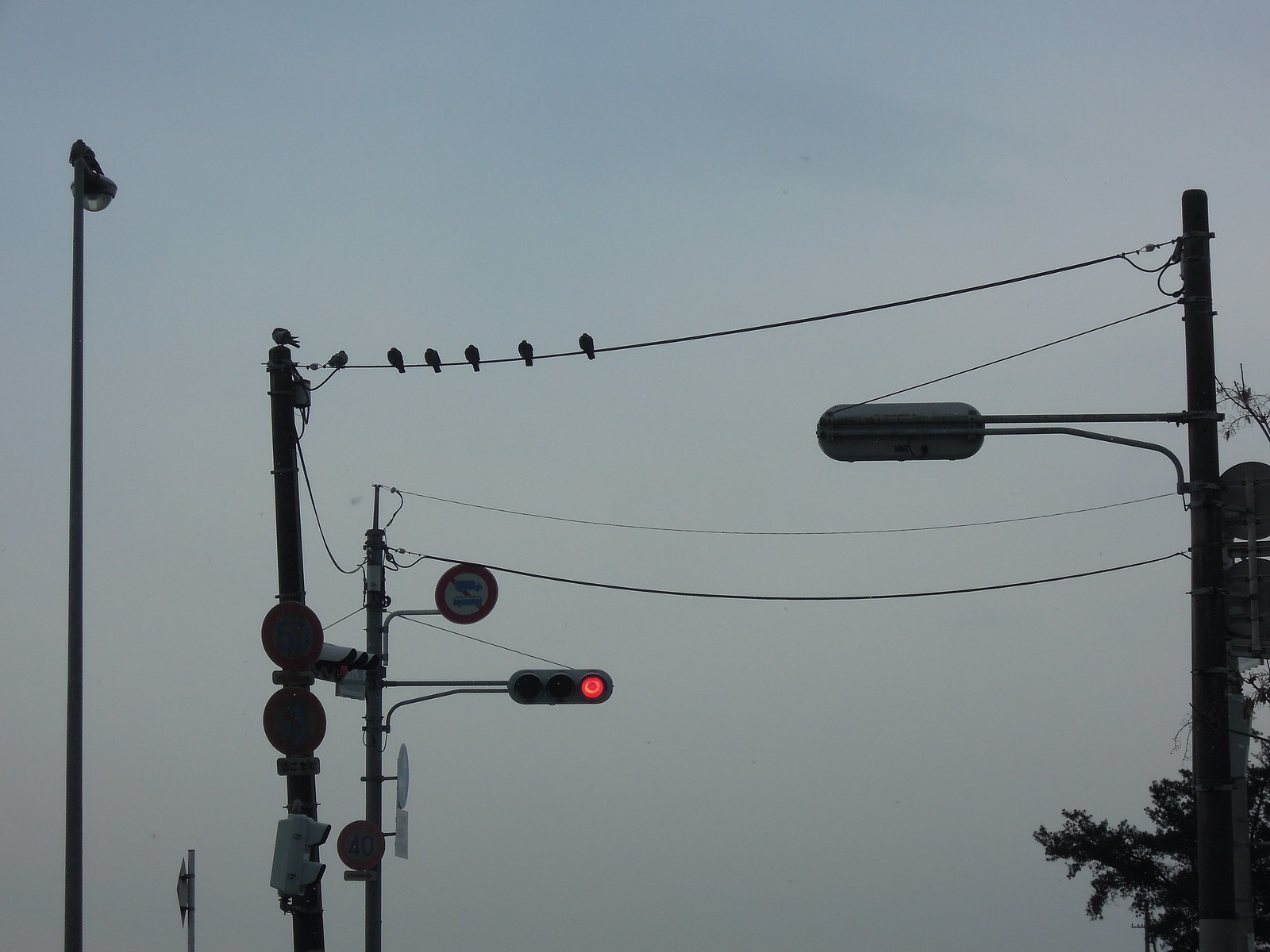This image captures an early twilight or dawn scene with a darker blue sky as the backdrop. Dominating the foreground are utility poles and electric lines running horizontally. Near the left side of the image, close to a tall pole that stretches almost the entire height of the scene, a single bird perches atop the stoplight pole. Spanning from this left-side pole to another on the far right are several birds, six in total, aligned on one of the electric lines. These birds appear to be of the same species, creating a striking silhouette against the sky. Below the birds on the left side is a red and white sign featuring a partially obscured cross. The attached traffic light underneath this sign shows a red signal. On the right, a brightly glowing streetlight extends from the electric pole, adding an element of illumination. In the bottom right corner, the lush green canopy of a tree stretches slightly into the frame.